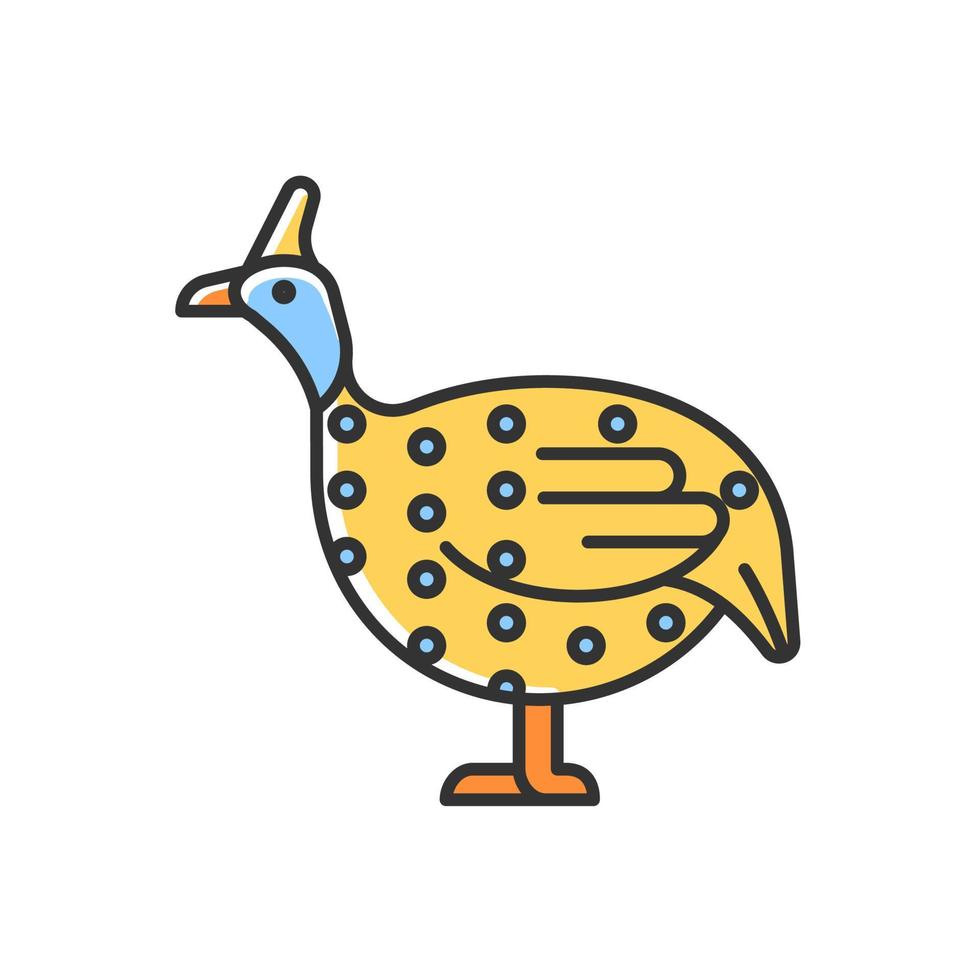This is a clipart-style illustration of a flightless bird resembling a chicken, duck, or turkey. The bird features a chubby, rounded yellow body adorned with bright blue polka dots, each outlined in black. It has an orange beak and orange feet, with a slight white layer visible on its underbelly. The head of the bird is blue, and it sports a yellow crest that matches the body’s coloration. The image is designed with thick black outlines for a simple, icon-like appearance. The background is plain white, highlighting the bird as the sole focus of the image.